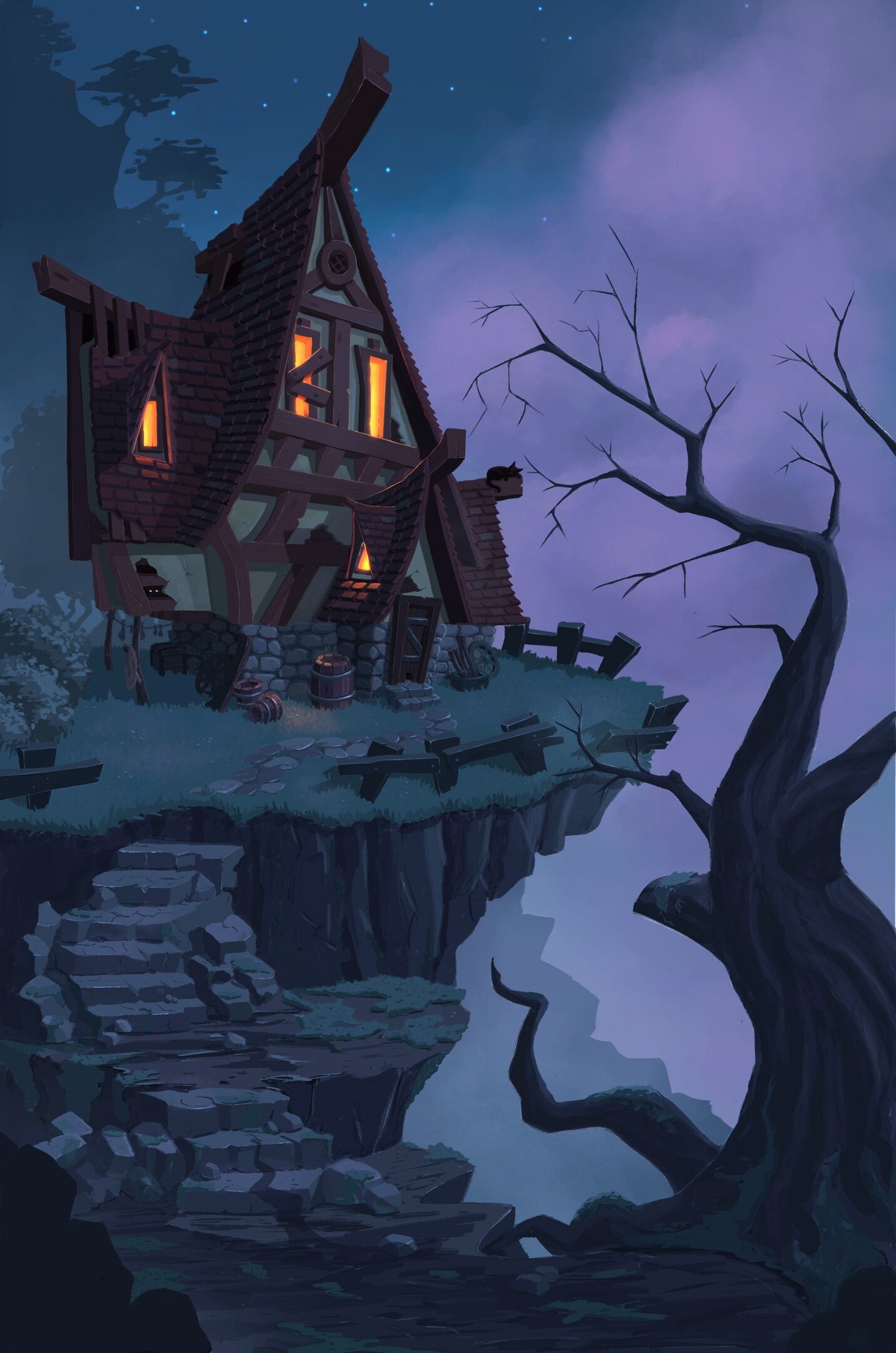This image is an intricate, computer-generated or animated depiction of a haunting yet cozy scene. Set against the backdrop of a star-lit night sky partially obscured by a thick fog, the scene reveals a towering, eerie, dead tree on the right, its sinister, curving branches pointing ominously towards a cliff edge. The tree's gnarled roots grip the rocky terrain of a steep cliff, accentuated by cracked stone steps winding up towards a plateau.

Atop the plateau sits a charming, triangular-shaped cottage that exudes both a mystical and inviting aura, perhaps the abode of a whimsical wizard. The house features a brown roof and walls adorned in green and wooden brown hues, standing on a sturdy stone foundation. From the four windows of the cottage, a warm, orange-yellow glow emanates, hinting at a glowing lantern or cozy fireplace inside. Additionally, a barrel is stationed beside the house, and a small fire flickers outside, contributing to the ambiance.

The entire scene, while imbued with elements of spookiness—such as the precarious rocky path and the insecure-looking fence—also offers a peculiar sense of warmth and homeliness. The silhouetted mountain in the distance further amplifies the dramatic and picturesque quality of this enchanting, animated landscape.